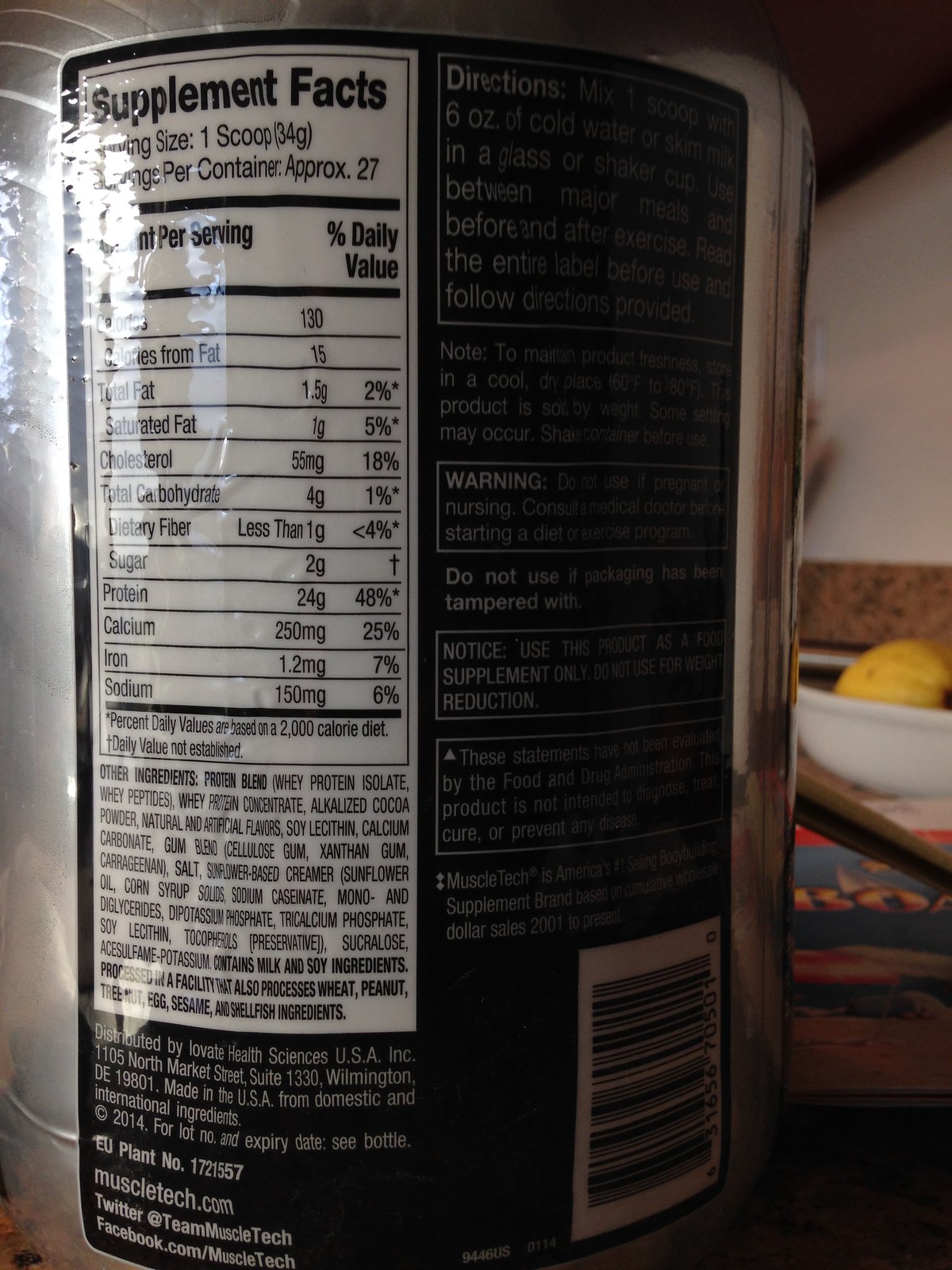The image depicts a close-up of a round, silver container labeled with detailed nutritional information and warnings, commonly associated with weightlifting supplements. The label predominantly features a black background with white text and includes sections detailing the supplement's ingredients, serving size (notably one scoop), and nutritional content, highlighting 130 calories per serving of a whey protein blend. Part of the label also features a white background with a barcode. The photograph is darkly lit, capturing a glare from an external light source on the upper left of the label. The scene is set on a countertop, with a book, a placemat featuring some text, and a white ceramic bowl with a banana visible in the background against a white wall.